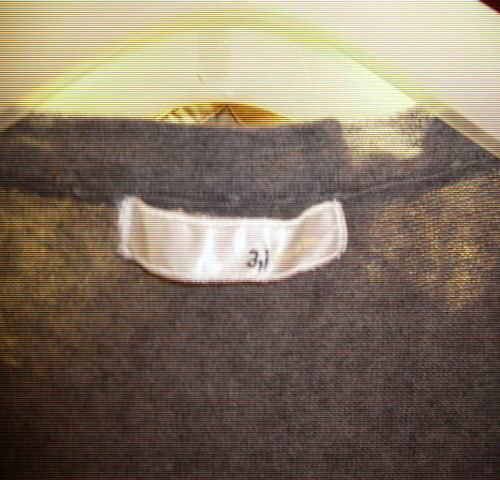This image showcases an extreme close-up of a piece of white fabric, which appears to be a clothing tag, layered over a brownish fabric background. At the top of the frame, there is a white, boomerang-shaped item, whose purpose is unclear. The background features a hint of gold, though its source is not identifiable. The brown fabric backdrop has distinct cutouts on the right side, revealing lighter, almost white patches beneath. The white fabric in the foreground prominently displays the letters "HE" in brown or black text. The overall composition of the image, with its zoomed-in focus, creates a sense of ambiguity, making it difficult to discern the exact nature of the objects featured.